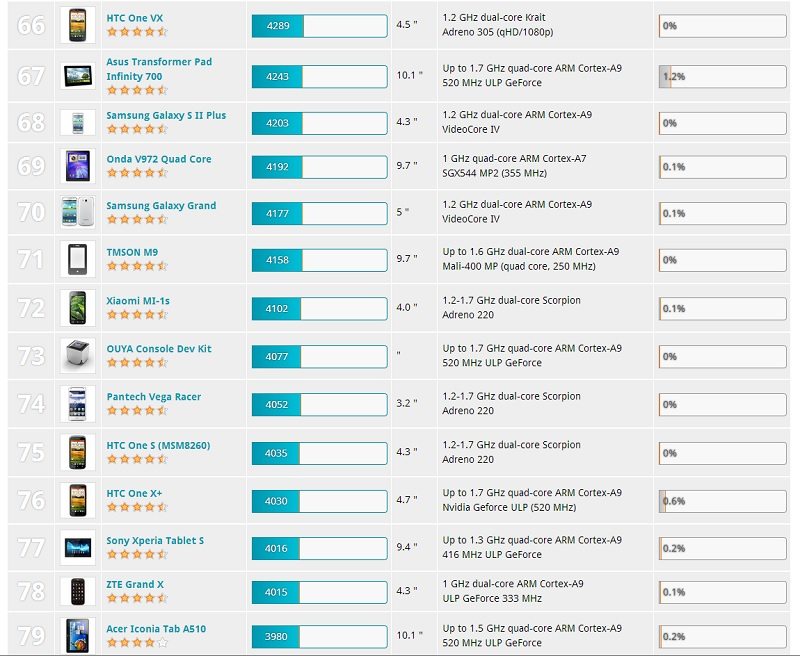The image is a vertical rectangular chart with no header, featuring a light gray background and divided into five columns. This detailed table seems to list and compare various electronic devices, likely smartphones or tablets, as indicated by corresponding images next to each entry.

- The first column on the left contains a sequential number pattern starting from 66 and ending at 79.
- To the right of each number, there is an image representing each device, which include models such as the HTC One VX and the ASUS Transformer Pad Infinity 700.
- Adjacent to the images in the second column, each device name is listed vertically.
- Below each device name, a series of stars likely indicate the review rating for each device.
- The third column consists of numbers in descending order displayed within blue boxes with white text, starting at 4289 for the number 66 and ending at 3980 for the number 79.
- The fifth column provides statistics specific to each listed device, though the exact nature of these statistics isn't specified.

Overall, this chart appears to be a comparative table of mobile devices, organized by ranking, images, names, review ratings, some numerical data, and additional descriptive statistics.